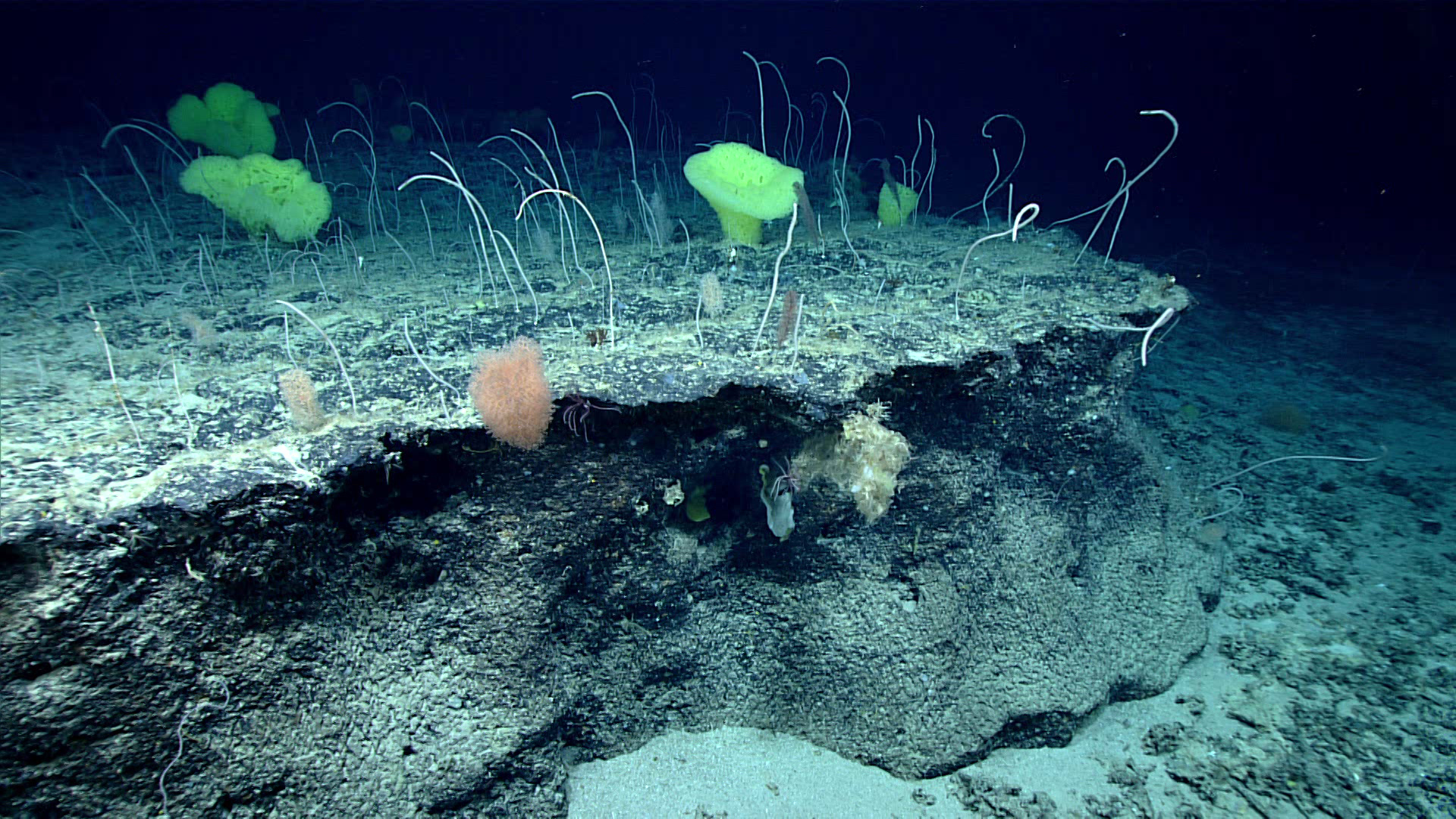This underwater photograph captures a vividly clear scene at the ocean floor, dominated by a large rock formation in the center. The base of the image showcases a light blue, sandy seabed interspersed with smaller rocky areas. The central rocky shelf has a face colored in darker, shadowed hues, while its upper surface shines light turquoise. A striking feature on this rock is the light yellow growth, possibly algae, covering parts of it. Emanating from the top are long, white, stringy structures reminiscent of worm-like shapes or hooks. Additionally, the rock hosts several bright green, mushroom-shaped corals and a couple of reddish-pink fuzzy blobs on its side. Throughout, there are green sponges and scattered sandy patches, with the background shrouded in deep navy blue darkness, highlighting the illuminated central rock formation against the shadowy depths of the ocean.